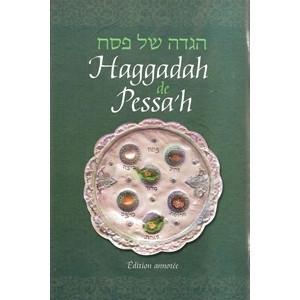The image displays the cover of a green book with foreign text, potentially Hebrew, prominently featuring "Haggadah de Pessa'h" in lighter green and white lettering at the top. Central to the cover is a detailed illustration of a white, scalloped-edged plate adorned with six colored circles, possibly representing symbolic foods. This plate appears to be an artifact or significant item in Hebrew tradition. The bottom of the cover indicates an edition of the book, though the specific wording is unclear.